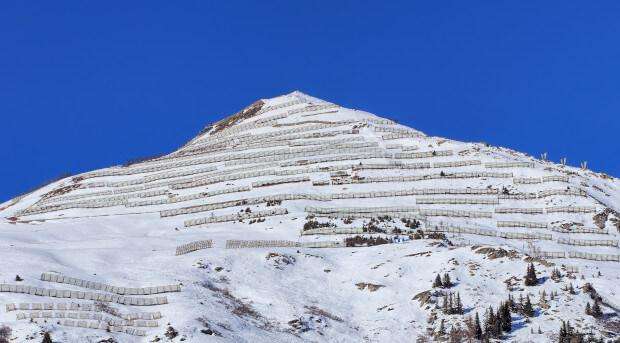In this striking photograph, the central peak of a snowy, white mountain dominates the scene, set against a vivid, royal blue sky. The mountain is crisscrossed by a series of brownish-tan mesh fences that stretch horizontally across its face from summit to base, most likely serving as snow barriers to prevent avalanches. Red flags are visible at intervals, likely marking a slalom route for skiers descending the mountain. Sparse pine trees dot the landscape, with a few concentrated in the lower right section of the image. The contrast between the bright snow, dark rocky patches, and strategically placed fencing creates a mesmerizing and practical panorama of a winter sports haven.